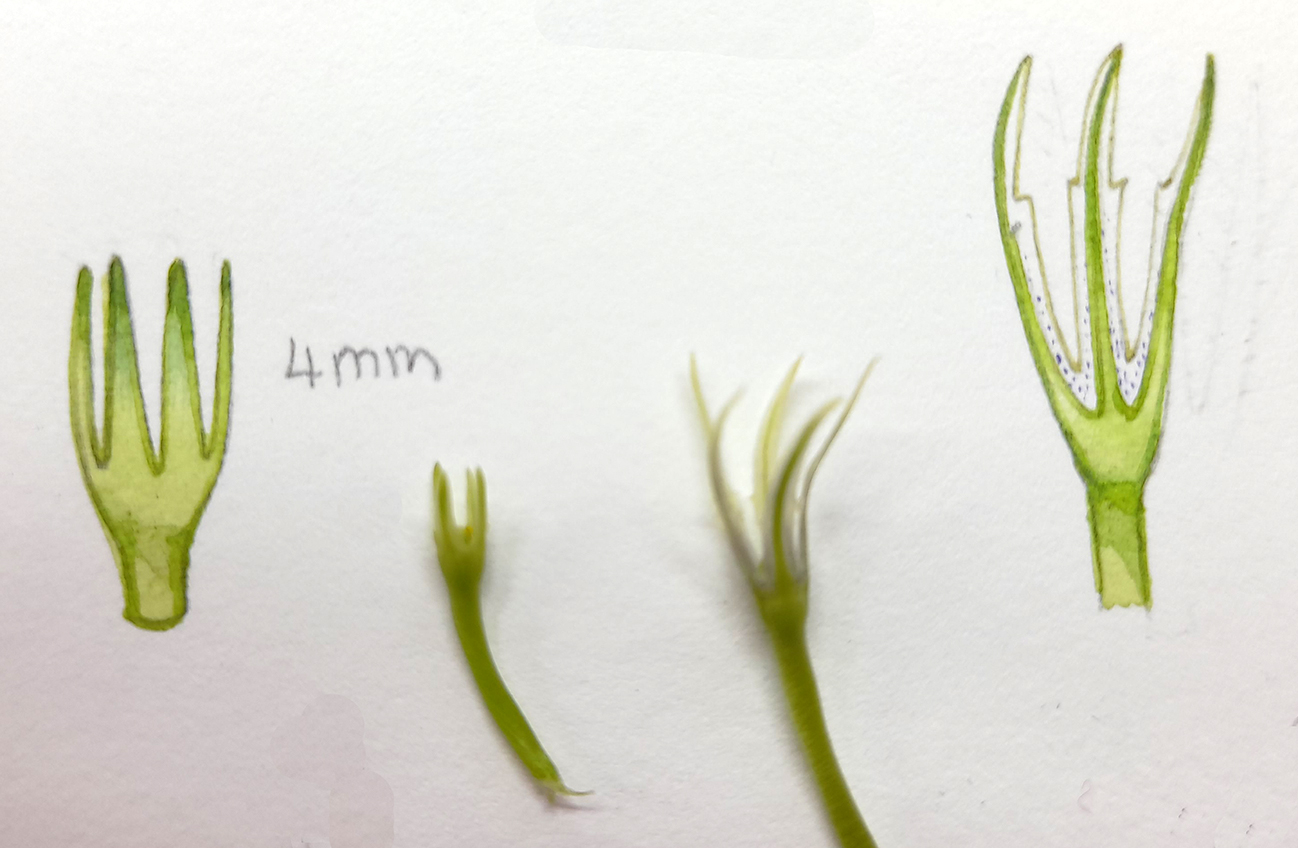This photograph showcases a detailed comparison between illustrated and real plant branches on a white paper background. On the far left, there's a meticulously drawn green plant segment with four forks at the top and a handwritten annotation that says "4mm," resembling a tall crown. Next to it lies an actual small plant piece, echoing the same structure. Adjacent to this is another real plant segment, slightly larger and spikier, featuring five or six forks. On the far right, the image is concluded with another drawing, depicting the plant with three forks. The arrangement presents a clear sequence: the first and fourth items are drawings, while the second and third are real plant pieces, providing a comprehensive depiction of the plant's varying forms.